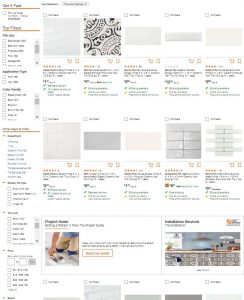The image depicts a close-up view of an assortment of tiles arranged in various configurations. The tiles vary in shape and size, including large and small square tiles, rectangular tiles, and ones about the size of a thick cigar. The colors predominantly range from cream to shades of gray, with hints of peachy and pink hues. Among the collection, there's only one tile with a repeating pattern, while the rest are either plain or feature unique designs. Some tiles showcase intricate arrangements, such as groups of three tiles aligned vertically on each side with a large tile bridging the top. The display aims to demonstrate different tiling patterns and configurations, possibly as inspiration for a backsplash project. Accompanying the image is a reference to an instructional video that guides viewers on calculating the necessary amount of tile for a given area.